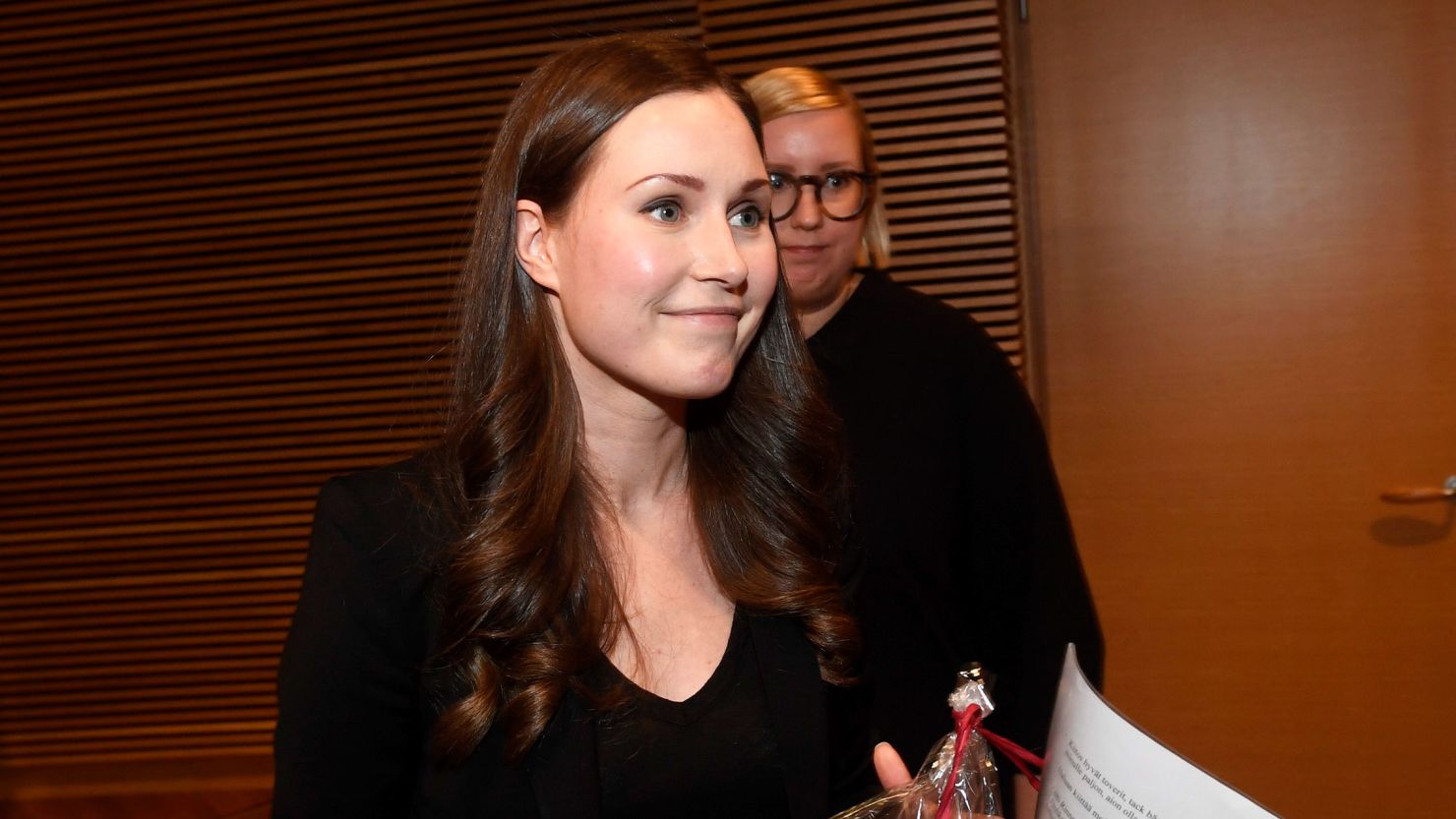This candid photograph captures two women standing in front of a large natural wooden wall and a redwood door with a visible handle. The photo appears to have been taken unexpectedly, as both women are looking off to the right of the frame, seemingly focused on something off-screen.

In the foreground stands a white woman, approximately 35 years old, with long brown hair that flows past her shoulders and is curled at the bottom while straight at the top. Her hair is parted in the middle, and she has green eyes, brown eyebrows, and a smile that suggests she might be reacting to something odd or surprising. She wears a black V-neck t-shirt paired with a black coat, revealing a hint of her cleavage. She holds some flowers and a few papers in her hands, adding an element of curiosity to her pose.

Behind her is another woman with chin-length blonde hair and large, black-rimmed glasses. Although her eye color is indiscernible behind the glasses, they appear dark. She is dressed in a long-sleeved black sweater and stands slightly more solemnly, also looking off-camera to the right. The image captures a moment of intrigue, framed by the natural wood paneling and the redwood door in the background, adding a rustic touch to this candid and detailed shot.